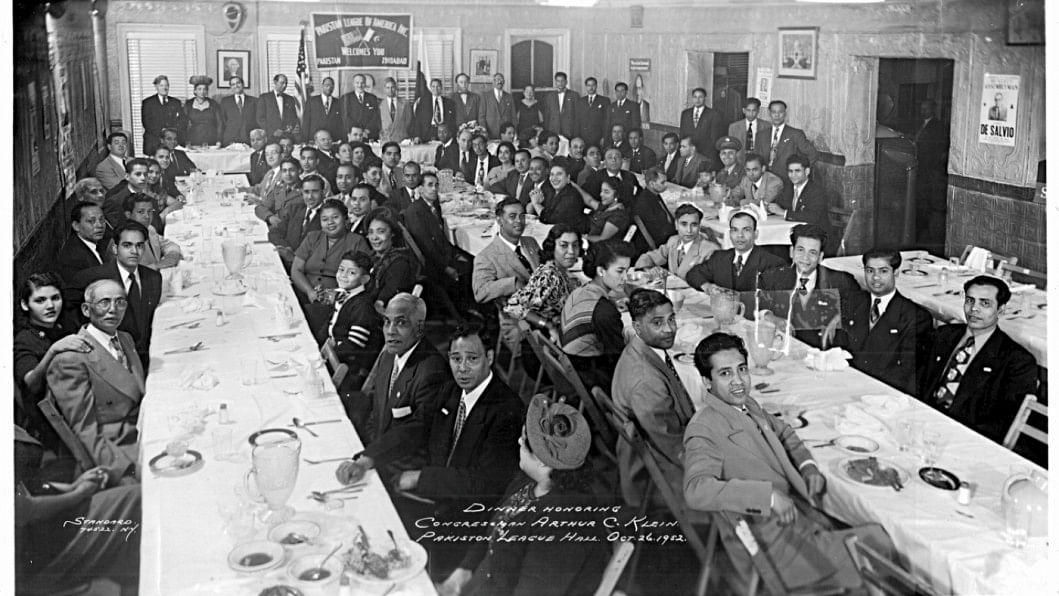This black-and-white photograph, taken on October 26, 1952, captures a formal dinner event honoring Congressman Arthur C. Klein at the Pakistan League Hall in New York, as indicated by the white script at the bottom. The image features a packed hall with three rows of long, narrow horizontal banquet tables that have been cleaned up, set with dinnerware, napkins, salt and pepper shakers, and drink pitchers. At the forefront, well-dressed men in suits and a few women in formal attire are seated, with children visible among them. Behind the diners, a head table or dais spans horizontally, with mostly men in suits standing, one of whom stands before an American flag. Paneled walls adorned with framed pictures surround the room, though the content of the frames is not clearly legible. The overall scene suggests a mid-20th-century atmosphere with a Filipino and Pakistani heritage gathering, reflecting the attire and ethnic makeup of the attendees.